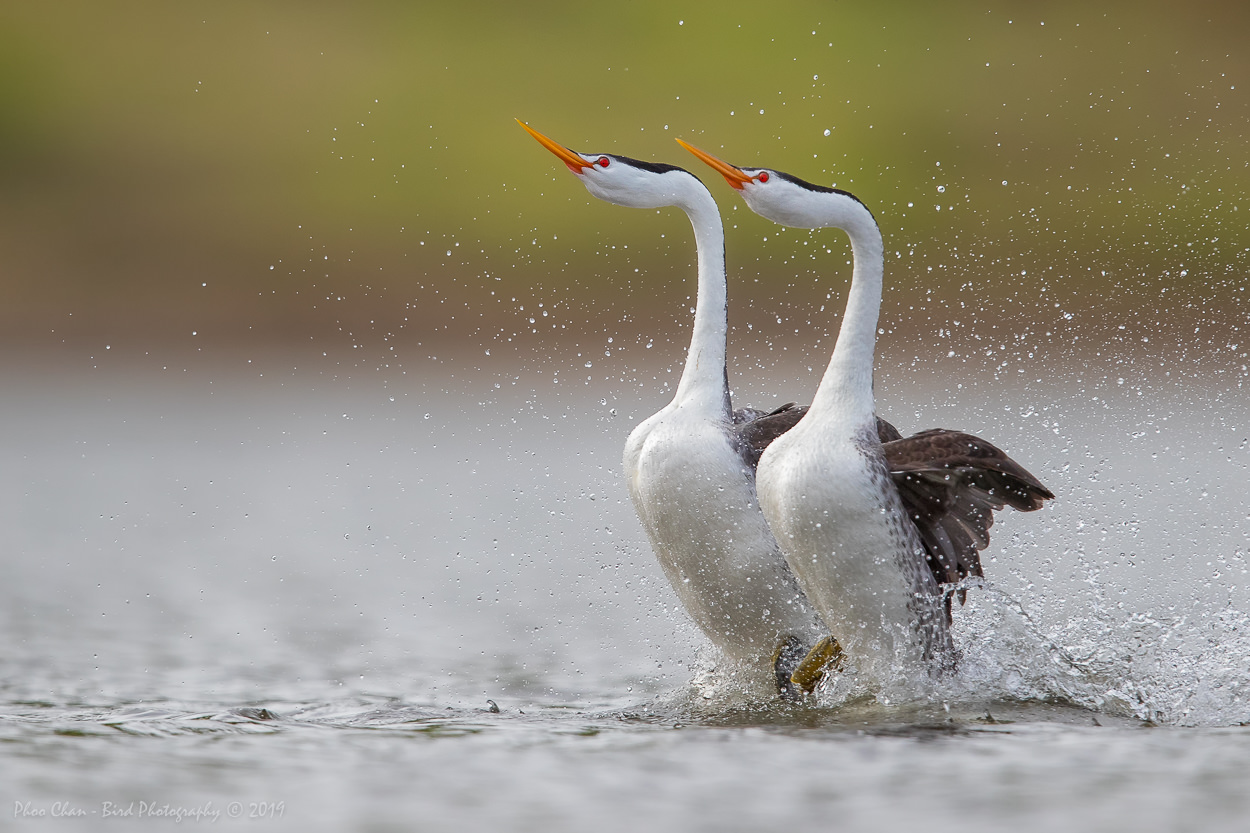This is a detailed and realistic photograph taken outdoors, oriented as a horizontal rectangle. The background is soft-focused in shades of light green and brown, hinting at trees and dirt, while the foreground features a shallow body of water. Central to the scene, on the right side of the image, are two large, identical birds, either geese or swans, captured in the act of landing and splashing in the water. Both birds have striking red eyes, long, thin orange beaks, and the crown of their heads are dark gray or black. Their necks are stretched out upward, displaying their white throats and chests. The birds' wings and back feathers are dark gray or black. The birds are aligned side by side, with their beaks pointed toward the upper left, causing their left profiles to be prominently visible. The ripples and splashes created by their landing add dynamism to the scene. In the lower left corner, the image is marked with a white cursive text that reads "Faux Clan Bird Photography © 2019."